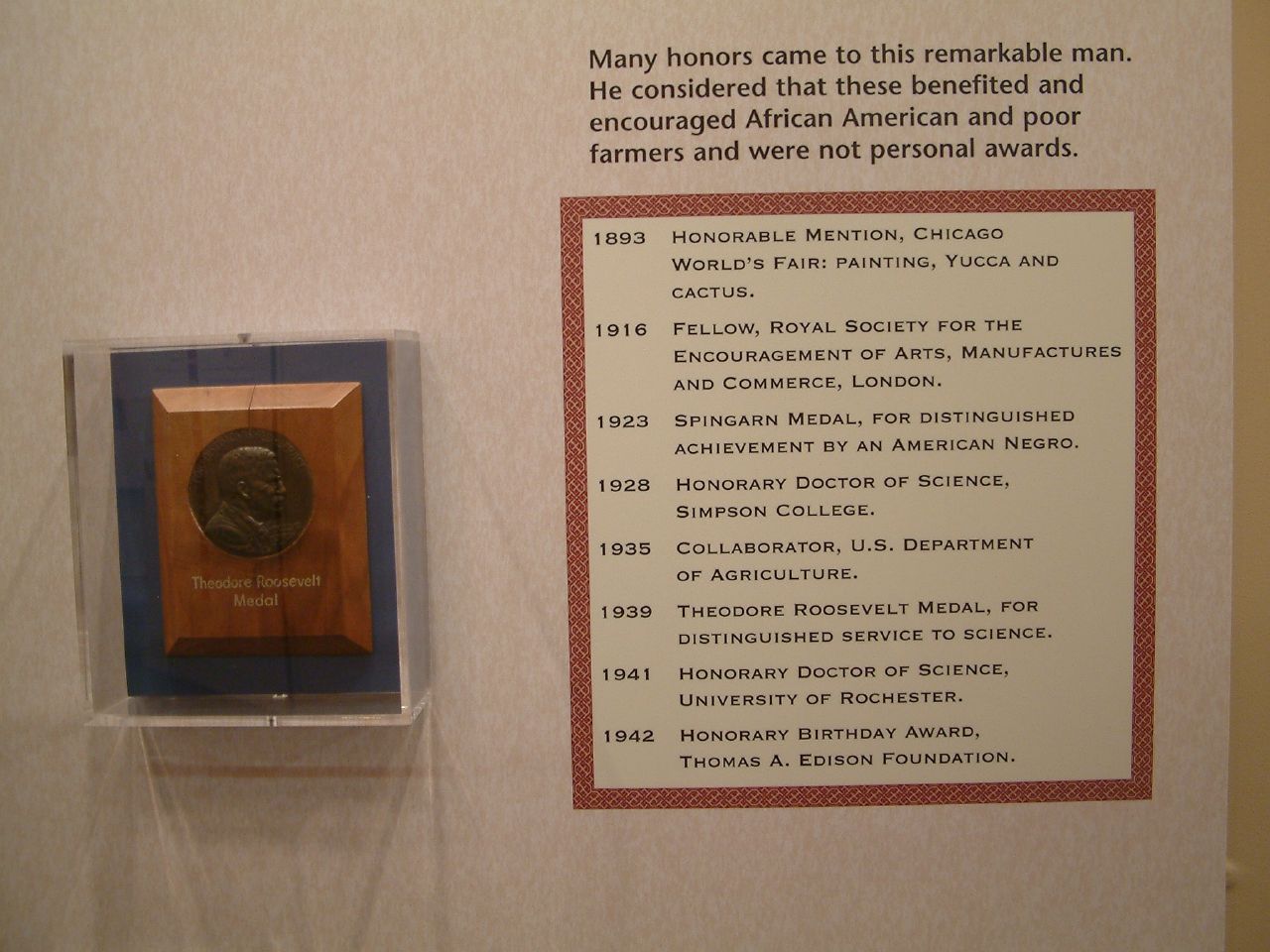The image depicts an exhibit, likely within a museum setting, dedicated to honoring a distinguished individual whose name is not explicitly mentioned. The exhibit is framed by a rich wooden wall with a notable bifurcation.

On the left side, encased behind glass, is a commemorative plaque made of polished wood. Embedded within the plaque is a bronze medallion identified as the Theodore Roosevelt Medal, inscribed with the medal's name below the emblem in gold font.

On the right side, the exhibit features an informational display in black font on the wooden background, reading: "Many honors came to this remarkable man. He considered that these benefited and encouraged African-American and poor farmers, and were not personal rewards." Beneath this text, within a bordered tan box with a red frame, a detailed list of awards and honors is shown, including:

- 1893: Honorable Mention, Chicago World Fair for the painting "Yucca and Cactus"
- 1916: Fellow, Royal Society for the Encouragement of Arts, Manufacturers and Commerce, London
- 1923: Spingarn Medal for Distinguished Achievement by an American Negro
- 1928: Honorary Doctor of Science, Simpson College
- 1935: Collaboration, U.S. Department of Agriculture
- 1939: Theodore Roosevelt Medal for Distinguished Service to Science (which is displayed in the glass case)
- 1941: Honorary Doctor of Science, University of Rochester
- 1942: Honorary Birthday Award, Thomas Edison Foundation

The exhibit clearly aims to highlight the numerous accolades received by this noteworthy figure, with a focus on how these honors served broader communities rather than personal acclaim. The colors visible in the image include tan, blue, brown, bronze, white, red, and black.